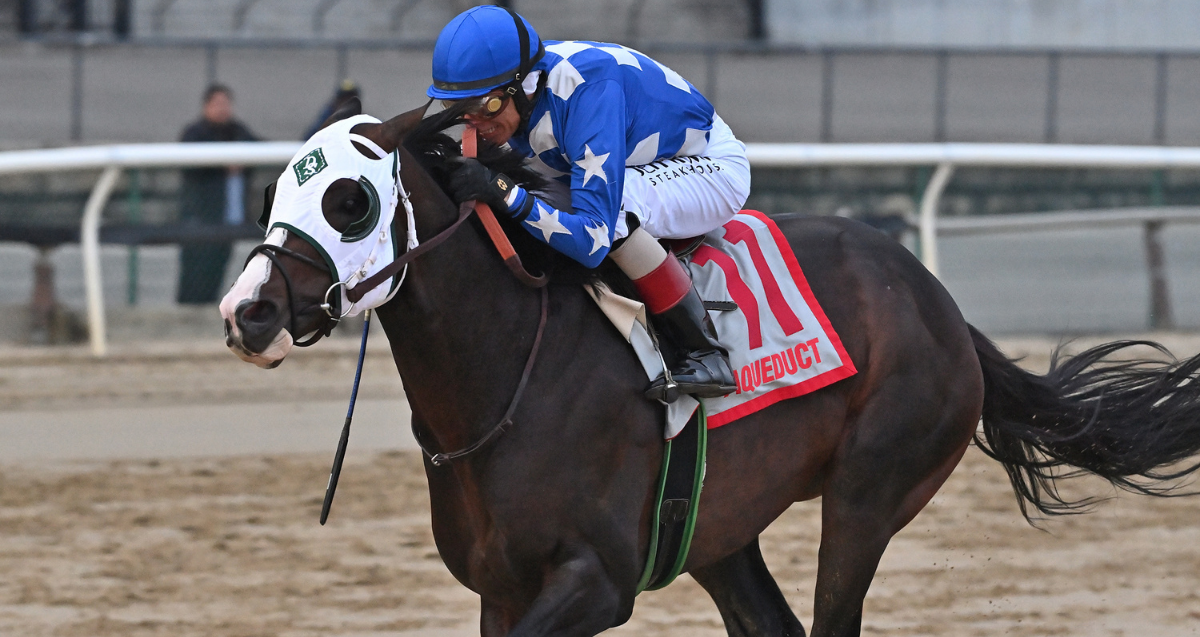In the image, a jockey clad in a blue cap and a blue shirt adorned with stars, accompanied by white pants and black boots, rides a dark brown racehorse. The horse is fitted with white blinders, featuring a distinctive triangle with the letter "G" on its forehead. The number 11 is prominently displayed under the saddle, with "Aqueduct" inscribed in red lettering bordered by a red outline. The scene captures the horse in mid-action, racing on a dirt track at Aqueduct Racetrack. In the background, there are distinctive racetrack fencing and a few spectators watching intently as the jockey strives to win the race.